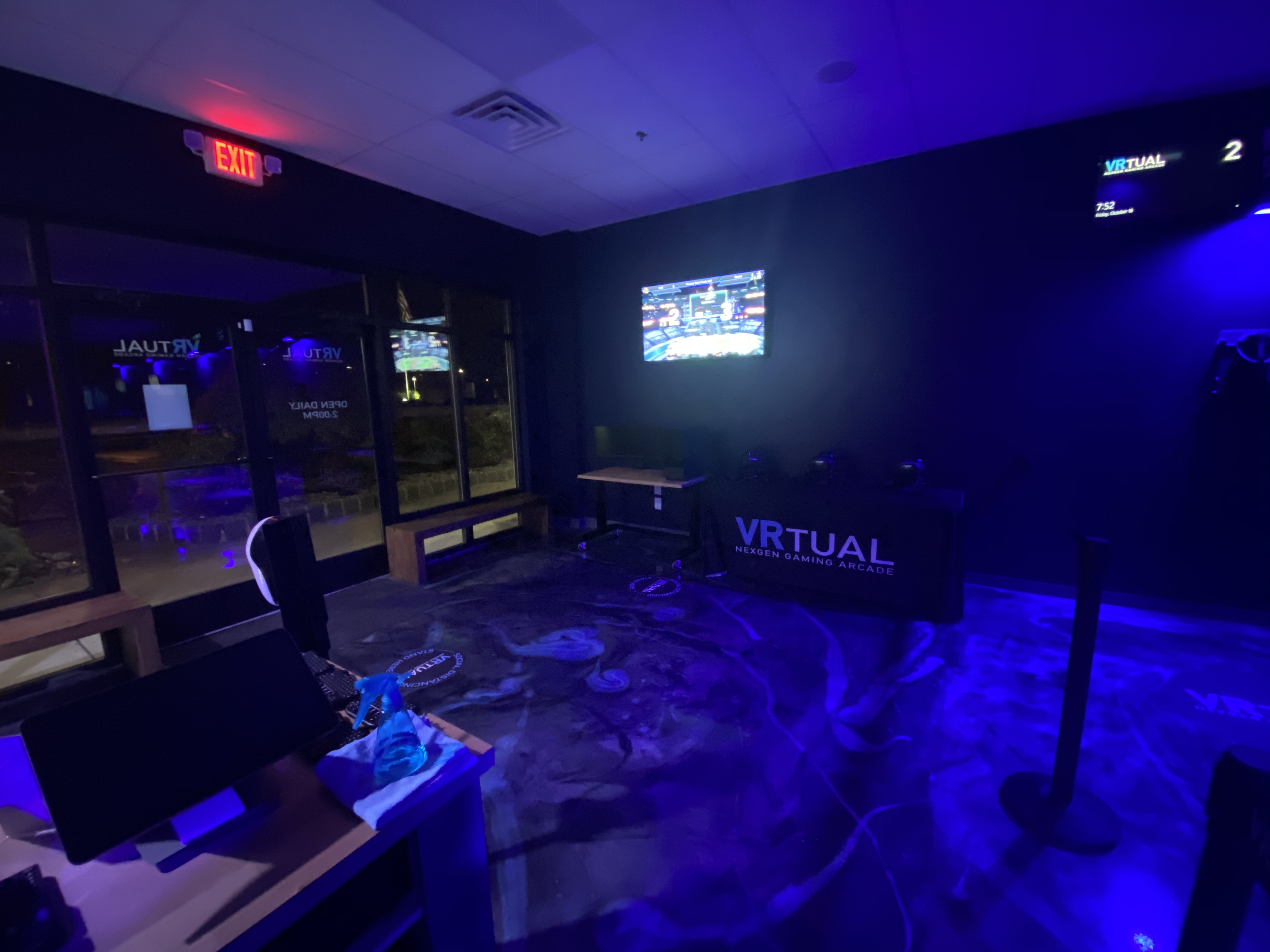The photograph depicts a dimly lit room with an immersive blue hue, likely a VR or game room. The left-hand side of the image showcases a series of large glass windows and a door, all reflecting the ambient blue light that fills the space. The ceiling, made of white tiles, also glows blue, enhancing the futuristic atmosphere. Mounted on one of the side walls are two illuminated screens, possibly TVs, with one displaying an image that suggests someone has just finished playing a game. Below these screens is a table draped with a cloth inscribed with the word "VIRTUAL." In the lower left corner stands a wooden desk with a dark screen on it, as well as what seems to be a computer setup. Wooden benches line the windows, contributing to the room's sleek and modern aesthetic.